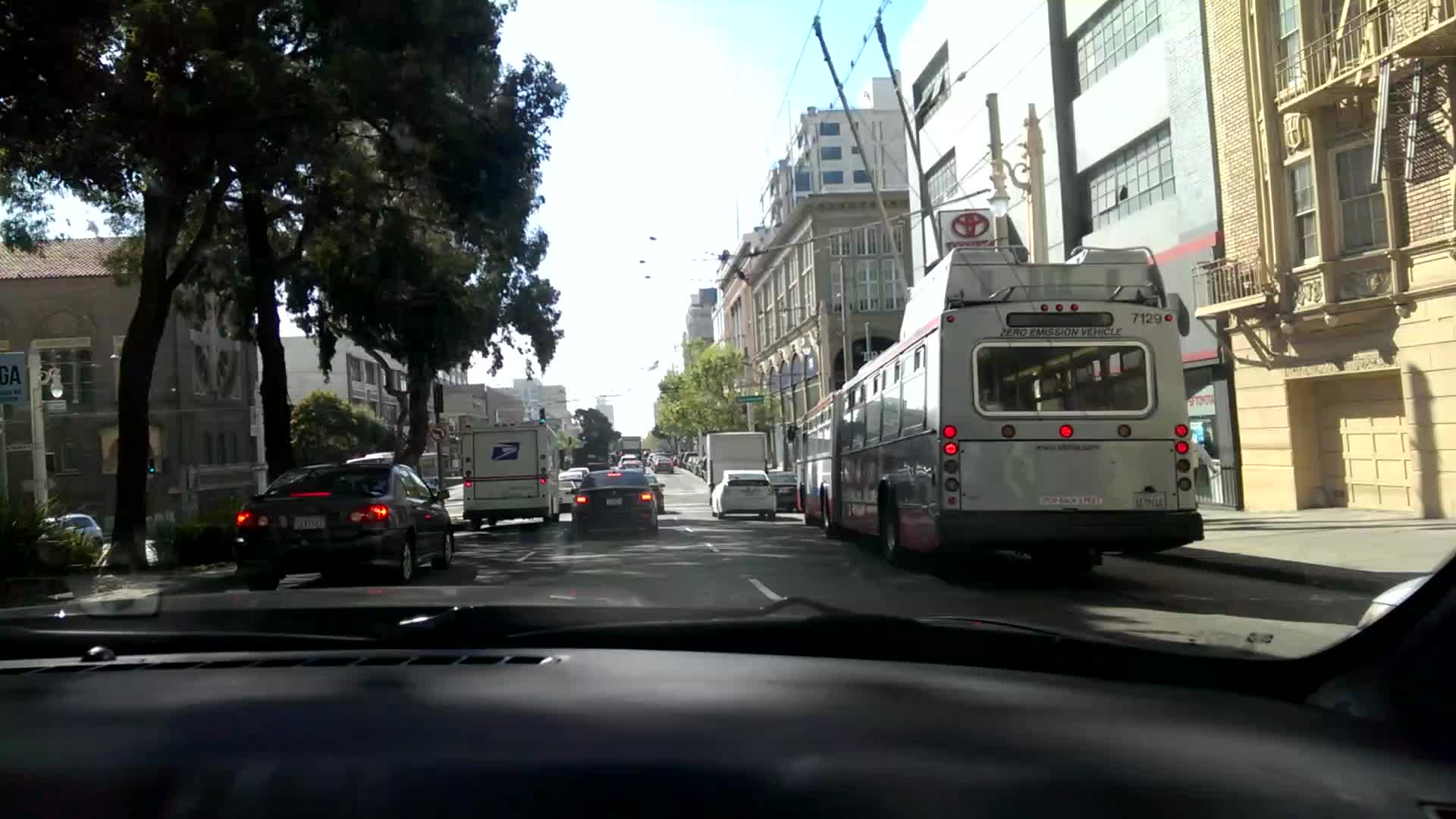The photograph, taken from inside a car from the passenger side seat, reveals a scene outside through the windshield, framed by the black dashboard and windshield edges. To the left, trees line the view, accompanied by a mix of shorter, grey buildings, indicating a smaller city or neighborhood devoid of towering skyscrapers. On the right, older buildings in shades of yellow, white, and grey create a vintage ambiance. Further in the distance, more trees can be seen.

The road ahead features multiple lanes, with at least three lanes visible going in one direction. In the central lane, a distinct mail truck is observable, flanked by several other vehicles, including a city bus. The overall scene depicts a bustling street with a blend of natural and urban elements, reflecting the character of an older, quieter part of a city.